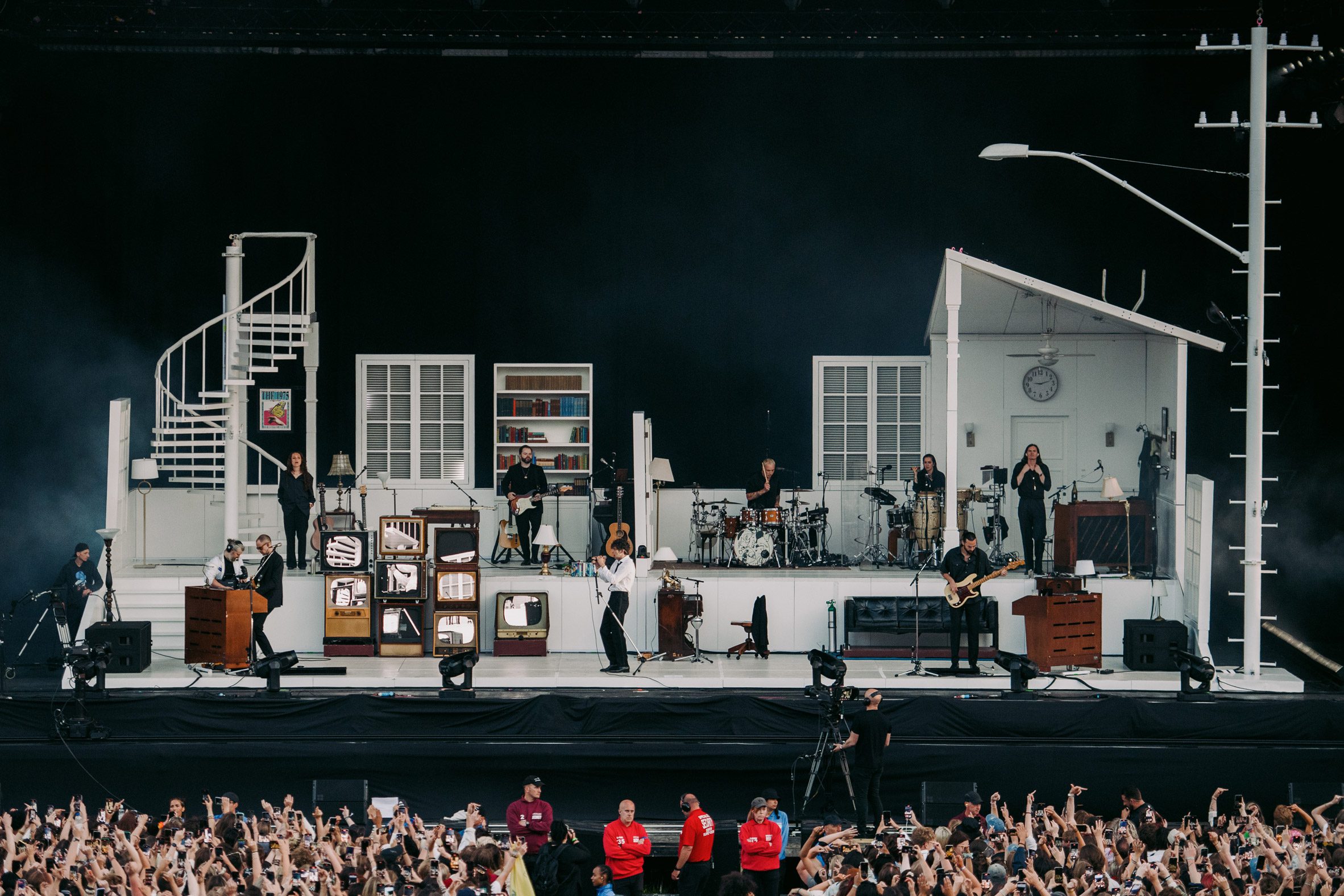The image captures an outdoor concert where the stage is intricately designed to resemble the interior of a house. The stage includes a lower platform with three guitar players and a keyboardist, and an upper level with two drummers and a vocalist. The setting features a white spiral staircase, a bookshelf filled with books, vintage TVs, windows, a black leather couch, and various other domestic decor pieces such as a house lamp and a clock. Performers are primarily dressed in black attire, though one man stands out without his coat. Among the instruments present are pianos, guitars, and drums. The audience, divided into two main groups on either side of the stage, energetically engages with the performance, many with their hands raised. In the midst of the crowd, three men wearing red shirts and others in maroon and light blue can be seen. A cameraman is also present to capture the event. The detailed ambiance of the stage along with the vibrant engagement of the audience creates a lively and dynamic scene.